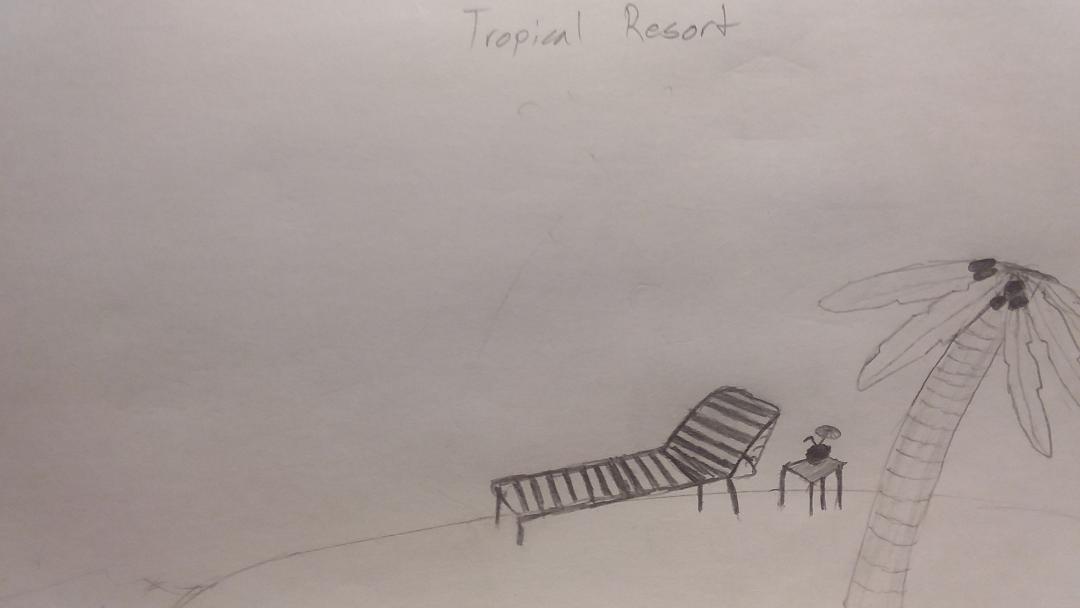This pencil-drawn illustration features a "Tropical Resort" theme displayed on a slightly wrinkled white sheet of paper. Subtle stray pencil marks and visible indentations lend an authentic, hand-drawn feel to the piece. Dominated by heavier pencil lines, a shadowed beach chair sits prominently in the center. To its side, a small table holds a tropical coconut drink, complete with a straw and a tiny umbrella. In the foreground, a meticulously detailed palm tree showcases individual lines etched along its trunk and distinct leaves above, with darkly shaded coconuts clustered at the top. The artist's crisp technique and attention to detail provide a captivating rendition of a serene beachside scene.